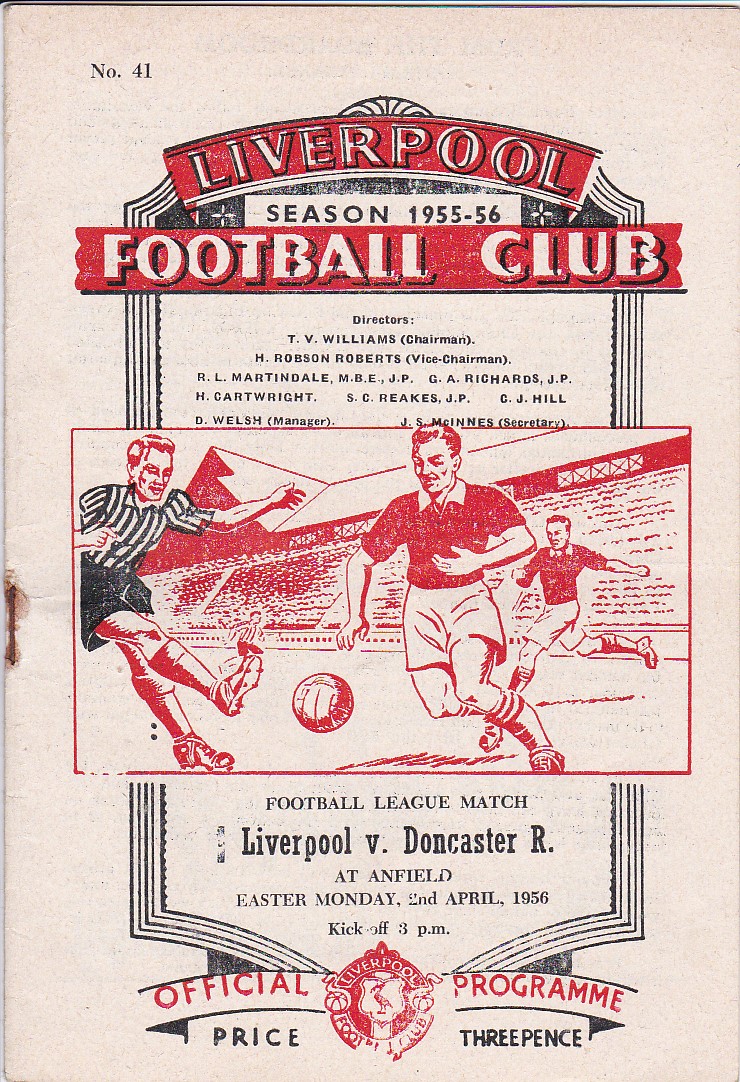The image is a rectangular, antique, official game day program from the Liverpool Football Club for the 1955-56 season, specifically issue number 41. The cover, now an off-white background with red and black ink, features a bold banner at the top reading "Liverpool" in a red background with black and white lettering, followed by "Football Club" beneath it. Between these banners is a smaller white strip stating "season 1955 to 56" in black text. Below the title, there's a section listing the directors of the club. Central to the cover is a hand-drawn illustration in red, black, and white depicting a football match in progress: three players mid-action—one kicking the ball, two others chasing it—with the referee, distinct in black stripes, overseeing the play, and the stadium stands filled with spectators in the background. The caption beneath the illustration announces the clash: "Football League Match Liverpool vs. Doncaster R at Anfield Easter Monday 2nd April 1956 kickoff 3 p.m." At the bottom, flanking the club's logo, the text reads "Official Program" with the price marked as three pence.